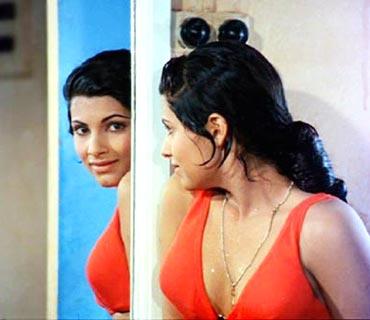In a nostalgic, film-like photograph that appears to date back to the 1960s, a young woman with long, dark brown hair, styled in a loose ponytail with some strands tucked behind her left ear, gazes thoughtfully into a mirror. Her reflection shows both the front of her softly smiling face and the side of her body, standing out subtly against a blue background seen in the mirror. The woman is wearing a salmon-colored top with a low V-neck cut, resembling a reddish-orange hue, and a silver necklace. The actual background of the room is a stark contrast of off-white, featuring a light fixture with two black bulbs visible above her. She is positioned on the right side of the photo, looking into the mirror on the left, capturing a serene and reflective moment from presumably her early to mid-twenties.